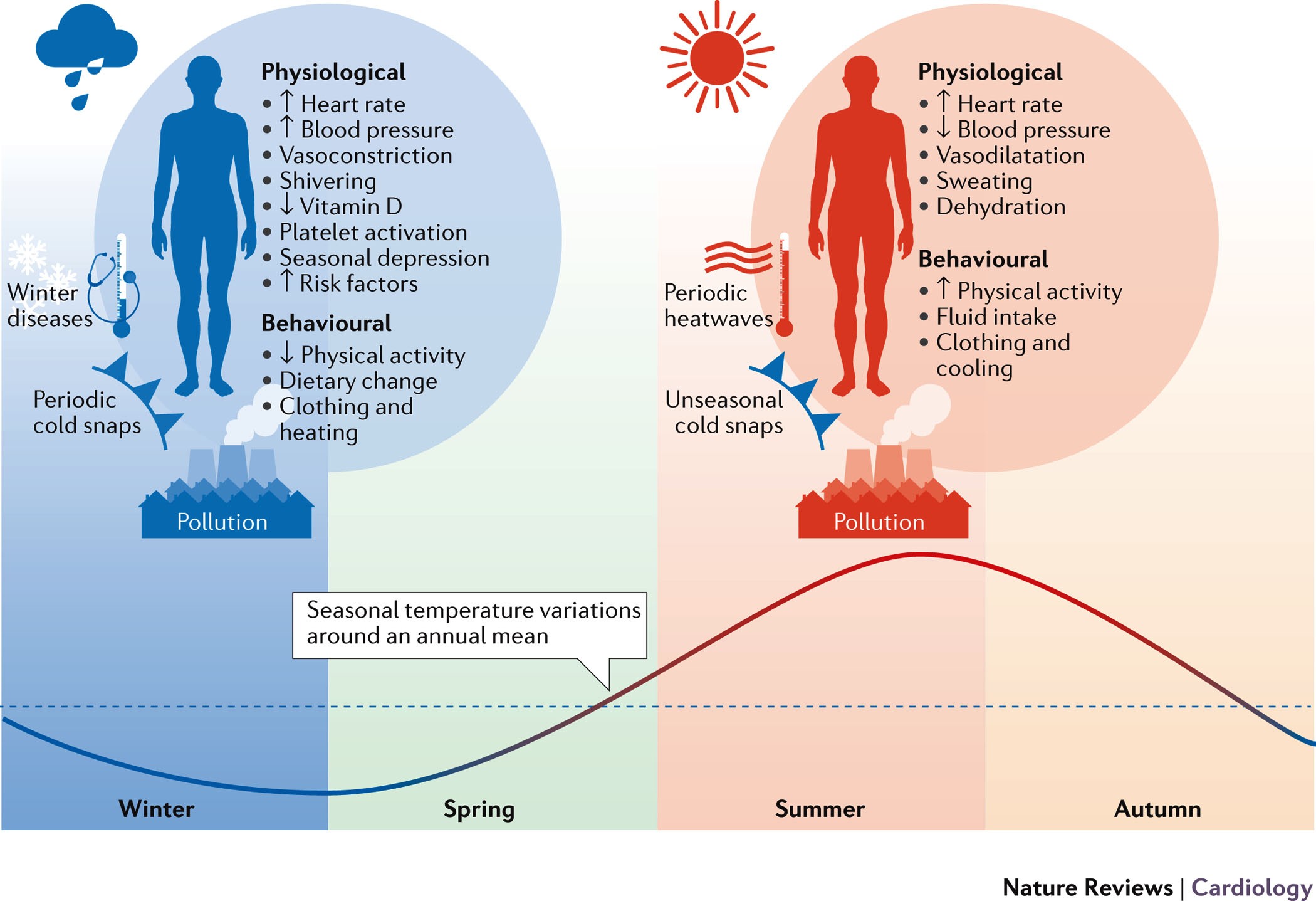This image, sourced from the textbook "Nature Reviews," focuses on cardiology and the impact of seasonal variations on cardiovascular health. The lower section of the image illustrates the four seasons: winter (blue), spring (green), summer (red), and autumn (pale orange). At the top, the image depicts two human figures representing different overlapping seasonal effects.

The winter and spring seasons are shown overlapping in shades of blue, highlighting physiological effects related to cold weather. Key details covered include:
- Periodic cold snaps
- Increased heart rate and blood pressure
- Vasoconstriction
- Shivering
- Decreased vitamin D levels
- Enhanced platelet activation
- Seasonal depression
- Elevated cardiovascular risk factors
Behavioral changes include reduced physical activity, dietary shifts, and adjustments in clothing and heating.

In contrast, the summer and autumn seasons overlap with a figure depicted in red, emphasizing the physiological and behavioral impacts of warmer weather. Important points mentioned are:
- Periodic heat waves and unseasonably cold snaps
- Increased heart rate, with blood pressure often decreasing
- Vasodilation and sweating
- Risk of dehydration
Behavioral adaptations include increased physical activity, heightened fluid intake, and changes in clothing and cooling mechanisms.

Additionally, the image acknowledges the role of pollution as a year-round impact affecting all seasons. Seasonal temperature variations around an annual average are highlighted, underscoring the potential changes in health dynamics throughout the year.